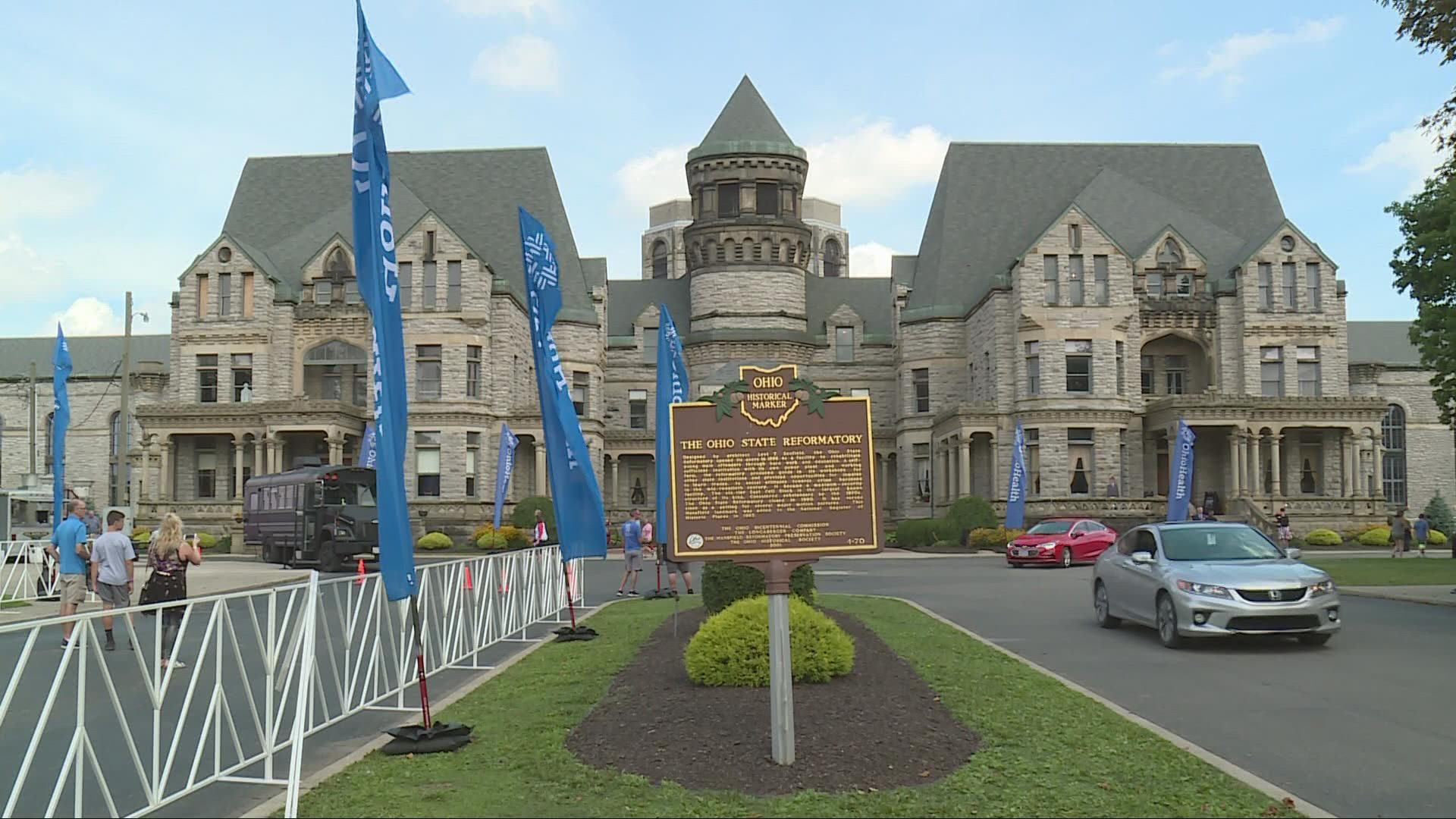The image depicts an outdoor scene featuring two large, gray buildings with numerous windows, connected by a central tower. These buildings appear to be part of a historical site. Between the structures, there is a prominent brown and gold sign that reads "Ohio State Reformatory" alongside an Ohio Historical Marker, though the smaller text on the sign is not fully legible. In the foreground, a well-maintained grassy area is bordered by decorative concrete, and a white fence adorned with blue ribbons and small flags runs along one side. Several cars are parked on an asphalt surface to the right, while a few people can be seen walking on the left. The scene is set under a light blue sky dotted with some clouds, suggesting a pleasant day.